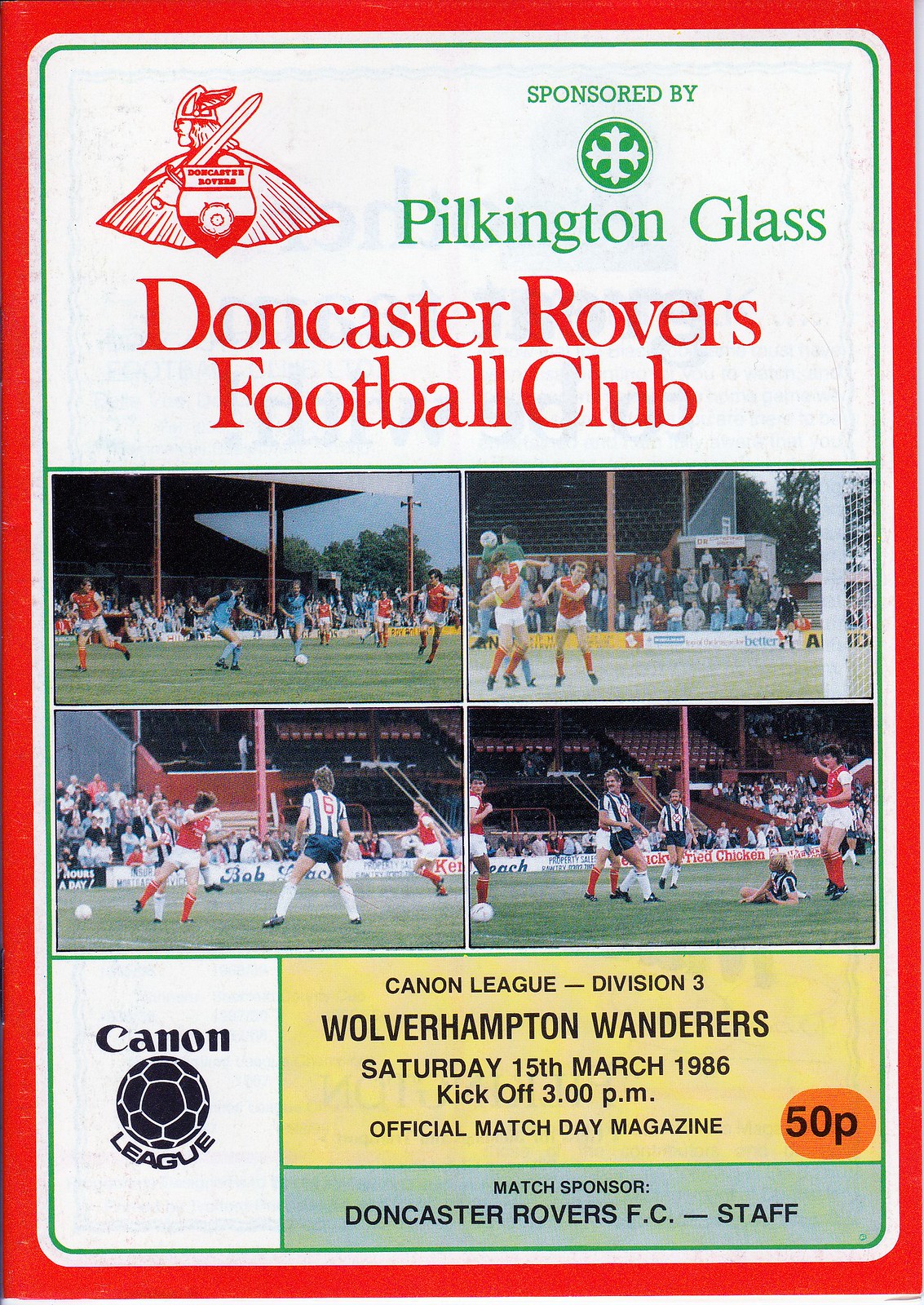This image is an advertisement for an upcoming football match featuring the Doncaster Rovers Football Club. The advertisement is set against a red background with a prominently outlined white section in the center. At the top of the ad, there is an emblem depicting a warrior or Viking holding a sword with a feathered helmet, set in a small shield-like icon.

The text at the top reads "Sponsored by Pilkington Glass and Green." Below this, the ad is divided into four smaller rectangular sections containing photographs of soccer action shots, arranged in two rows and two columns. Following these images, the text highlights the specifics of the match: "Canon League Division III Wolverhampton Wanderers, Saturday, 15th March 1986, kickoff 3 p.m.," clearly marking the game details.

The bottom left corner displays the Canon League logo alongside the match particulars. Additional information includes that this is the "official match day magazine" and the price marked by an orange circle with "50p." At the very bottom, a green box states "Match sponsored by Doncaster Rovers FC staff."

This thoroughly detailed advertisement effectively promotes the match, culminating in an eye-catching, informative poster adorned with historical football imagery.